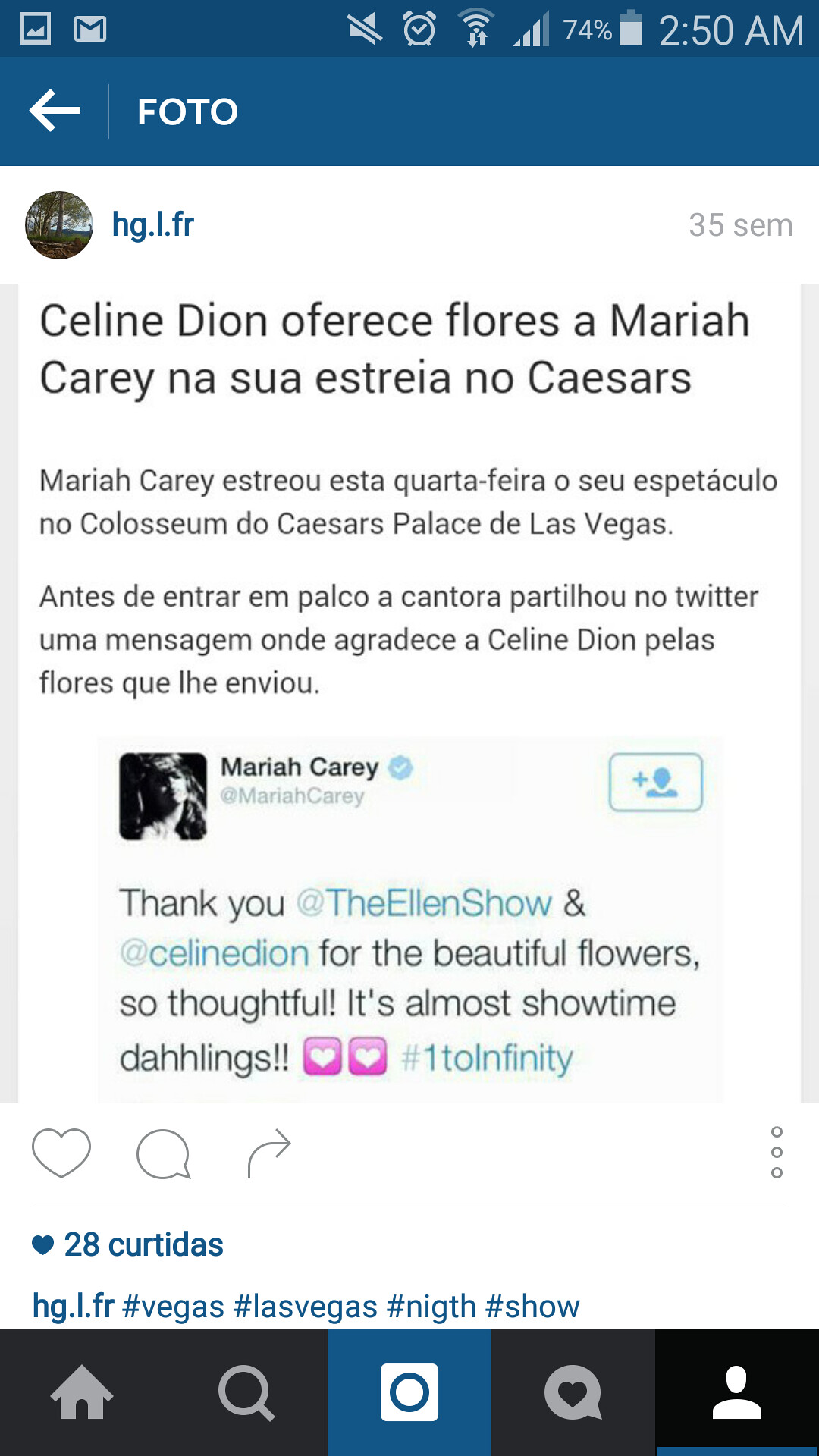The image is a screenshot taken from a mobile phone, displaying a Facebook post. At the very top, it features the phone's status bar in a blue rectangle with "photo" (F-O-T-O) on the left, alongside icons for Gmail, an alarm clock, a wireless signal, a 74% battery indicator, and the time "2:50 AM." The account posting on Facebook is "hg.l.fr" with an avatar of trees. The post itself is predominantly in Spanish, discussing Celine Dion sending flowers to Mariah Carey. It mentions “Celindian Ofrece Flores Mariah Carey Nasúa Estrella No Caesars” and further details about an event at Caesar's Palace in Las Vegas. Below this text, there's a retweet from Mariah Carey’s official account, verified by a blue checkmark, expressing gratitude to "The Ellen Show" and Celine Dion for the flowers, stating: "Thank you @TheEllenShow and @CelineDion for the beautiful flowers. So thoughtful. It's almost showtime darlings. ❤️❤️ #OneToInfinity.” This retweet garnered reactions from 28 users. At the bottom of the screen are navigation icons including home, search, and profile options, thereby indicating it was captured from a mobile phone interface.